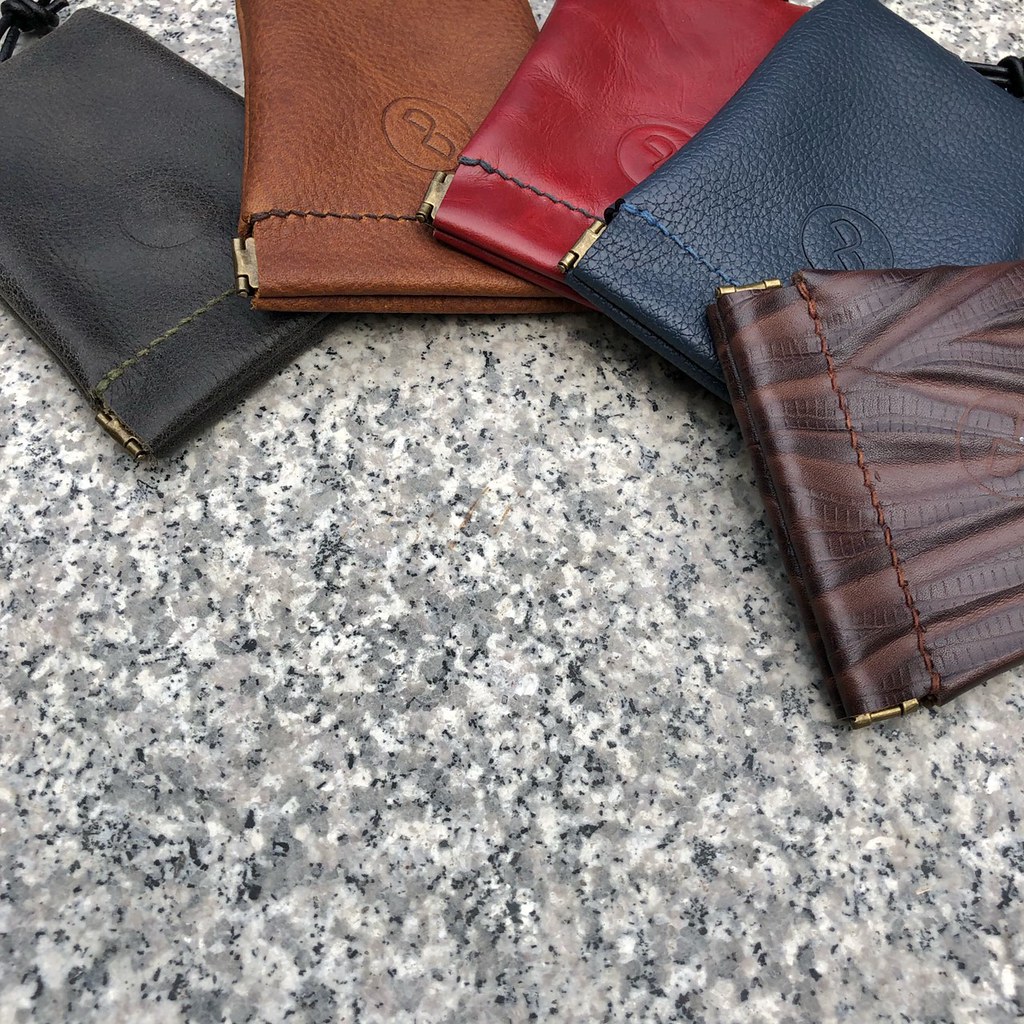The photograph is a color image showcasing five leather pouches, likely vintage cigarette cases, arranged in an arc on a granite countertop. The granite surface features a speckled pattern of dark gray, white, and black. The pouches come in various colors: dark brown, navy blue, red, black, and a multi-toned brown resembling exotic skin. Each pouch is adorned with a gold metal trim at the edges and bears a logo resembling a circle with the letters "DD" or the number eight inside. The pouches, which may open by pushing the sides together, were possibly used for cigarettes but might now serve purposes like holding phones or makeup. The scene appears to be lit under natural daylight, suggesting it could be a shop counter or display.